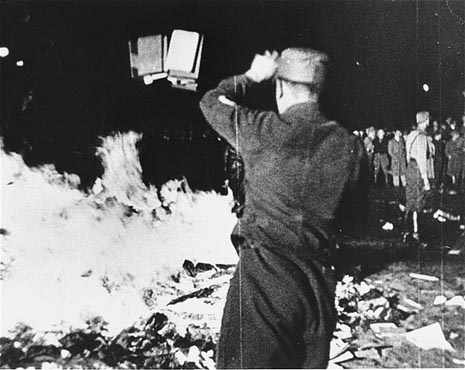In this black-and-white photograph, likely from the World War II era, a man dressed in dark pants, a dark shirt, and a tight-fitting cap is captured mid-action as he throws several books into a roaring fire that dominates the left side of the image. The scene is marked by a night-time setting, with a dark backdrop intensifying the flames. On the ground near the man, there is considerable debris and numerous books scattered about, suggesting they are also destined for the flames. To the right, a group of people stand and observe the spectacle, one of whom, potentially a soldier, is identifiable by his uniform and a strap across his chest, with his back turned to the camera. The photograph's splotchy quality and the clothing styles emphasize its historical context, reminiscent of the Nazi book burnings during WWII.